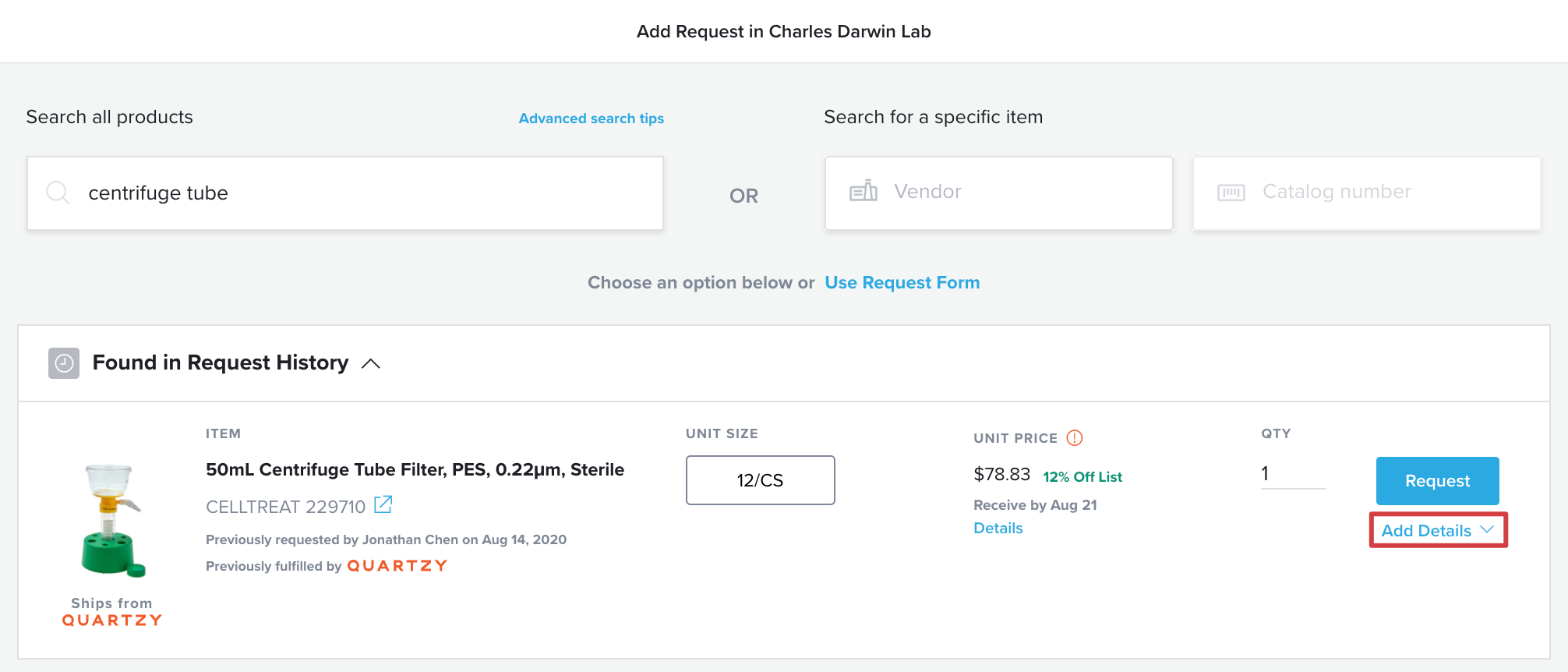Caption: 

In Charles Darwin's lab, a lab equipment search interface is displayed prominently. At the top, it features a light gray box labeled "Search All Products," accompanied by a white rectangular search bar with a magnifying glass icon and the text "Centrifuge Tube." Below, a blue area highlights an "Advanced Search" option, followed by a secondary search bar labeled "Vendor" and another titled "Catalog Number." Above these, it reads "Search for a Specific Item" with instructions below, stating "Choose an Option Below or Use Request Form."

Further down the interface, a white box displays items found in the request history. Featured prominently on the left is a 50 milliliter centrifuge tube filter with a green base, specified as "PES 0.22 µm Sterile Cell Treat." The item is noted to ship from Corsi.